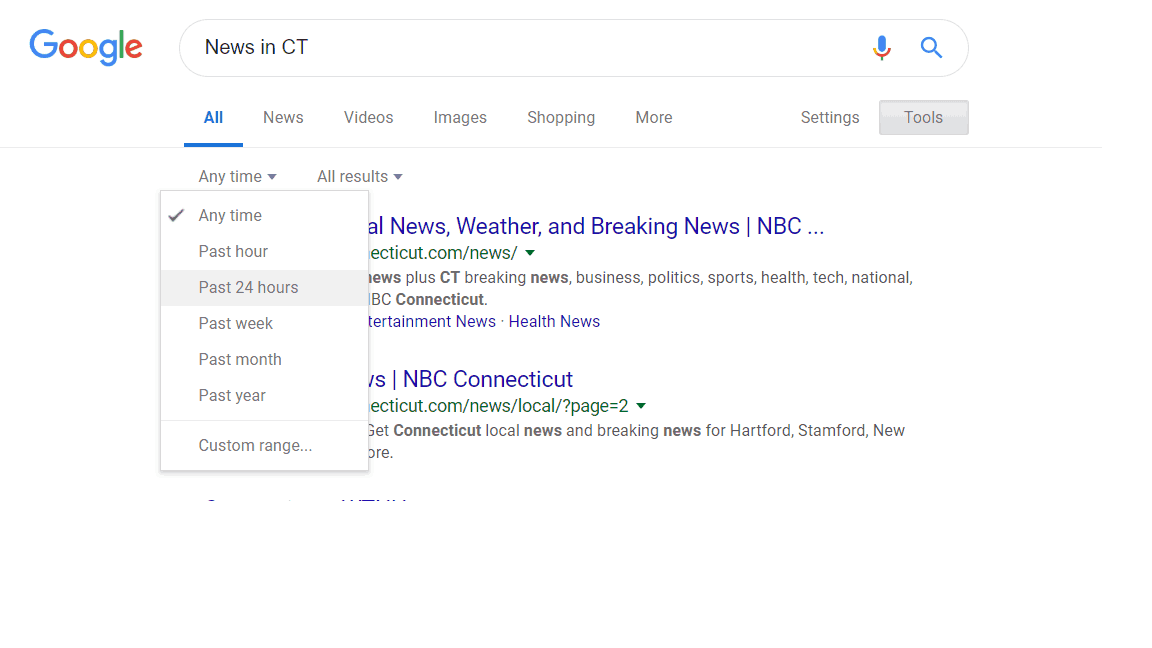The image shows a Google search results page with the recognizable Google logo featuring the colors blue, red, yellow, and green, positioned on the left side. In the search bar, the query "News in CT" is entered. The user has accessed the time filter menu, selecting "Any time," which is indicated by a check mark, while the "Past 24 hours" option is highlighted in gray.

The interface displays various Google search options, including "All," "News," "Videos," "Images," "Shopping," and "More," along with additional settings. Upon selecting the "Any time" filter, the dropdown menu obscures a portion of the search results. Below the search options, headlines such as "News," "Weather," "Breaking News," and "NBC Connecticut" are visible in blue headers, followed by green URLs and black body text.

The search results page also includes links to different categories like "Entertainment News" and "Health News." These links appear in blue. Above the results, next to the "More" option, are buttons labeled "Settings" and "Tools." The page predominately features a white background with mainly black text, accented by the blue and green hues of the links, adhering to Google's color scheme.